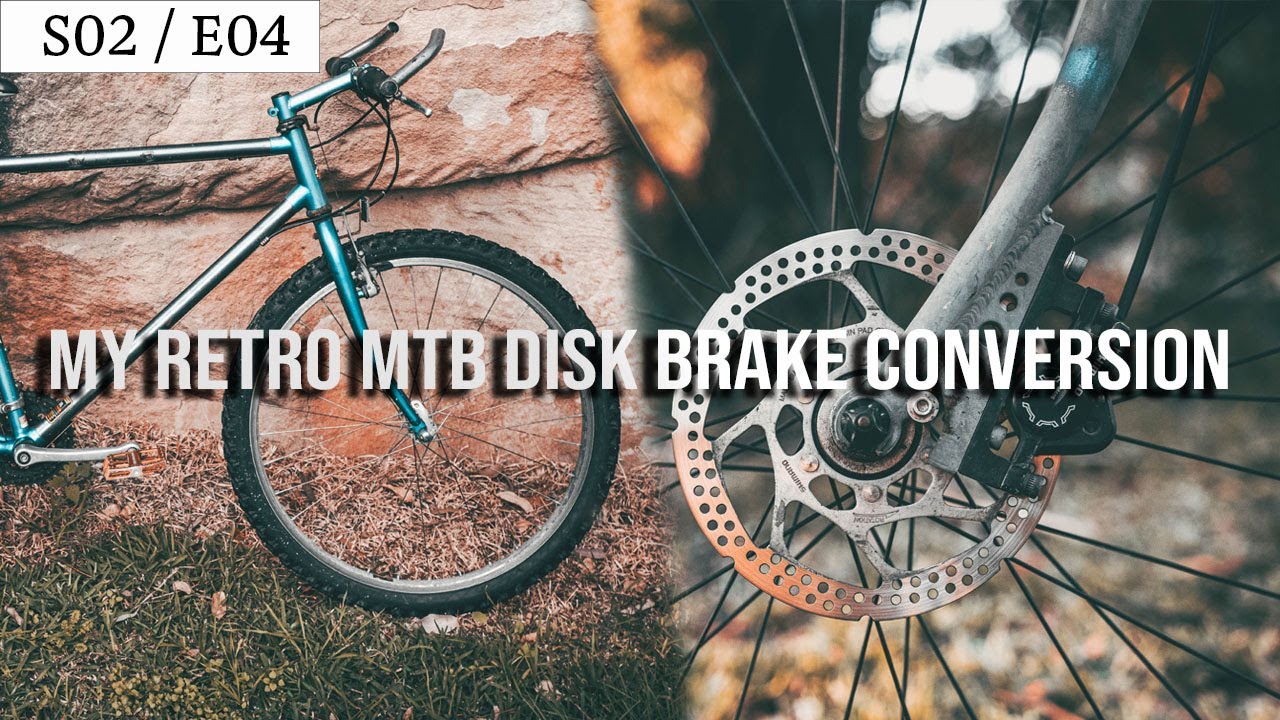The composite image features two distinct real-life photographs divided by a diagonal line at approximately a 45-degree angle. On the left side of the image is the front half of a bicycle, propped against a rugged rock wall with a grassy foreground. The right side showcases a close-up of a bicycle wheel's inner part, specifically the hub and spokes. This wheel includes a metal bracket and a circular disc, distinguishing it from the wheel in the left image. The background here is artfully blurred, featuring a bokeh effect with what appears to be fallen leaves. In the top left corner is a white rectangle containing black text that reads "S02/E04". Across the middle of the composite image, there is bold, all-caps sans serif text with a black shadow effect, stating "MY RETRO MTB DISC BRAKE CONVERSION".